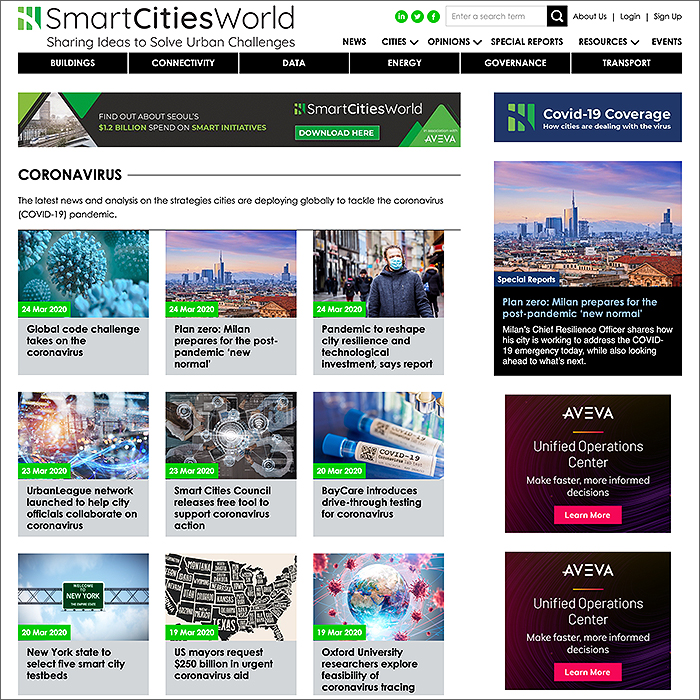This is a detailed screenshot of the Smart Cities World website as viewed on a computer. The website's logo is situated in the upper left corner, displaying "Smart Cities World" with "Cities" in bold black font and "Smart" and "World" in regular black font. To the right of the logo, there are three green social media buttons for Facebook, Twitter, and Instagram. Adjacent to these buttons is a search bar, and in the very upper right corner, there are hyperlinks for "About Us," "Login," and "Sign Up."

Just below these upper elements, a slogan reads, "Sharing Ideas to Solve Urban Challenges" in bold black letters. Further down is a navigational menu comprising drop-down options for "News," "Cities," "Opinions," "Special Reports," "Resources," and "Events." Following this, another row of clickable buttons is displayed, labeled from left to right: "Buildings," "Connectivity," "Data," "Energy," "Governance," and "Transport."

Beneath these buttons, a prominent banner announces, "Find Out About Seoul," highlighting that South Korea has invested $1.2 billion in smart incentives. The banner includes a call-to-action, "Smart City World, Download Here," and sponsors like Aveva. To the right of this banner, another banner features a section for "COVID-19 Coverage" with a subsection titled "Coronavirus" that offers the latest news and analytical analysis on strategies cities worldwide are employing to manage the pandemic.

Below this section, there are nine distinct boxes, each representing various plans for combating COVID-19.